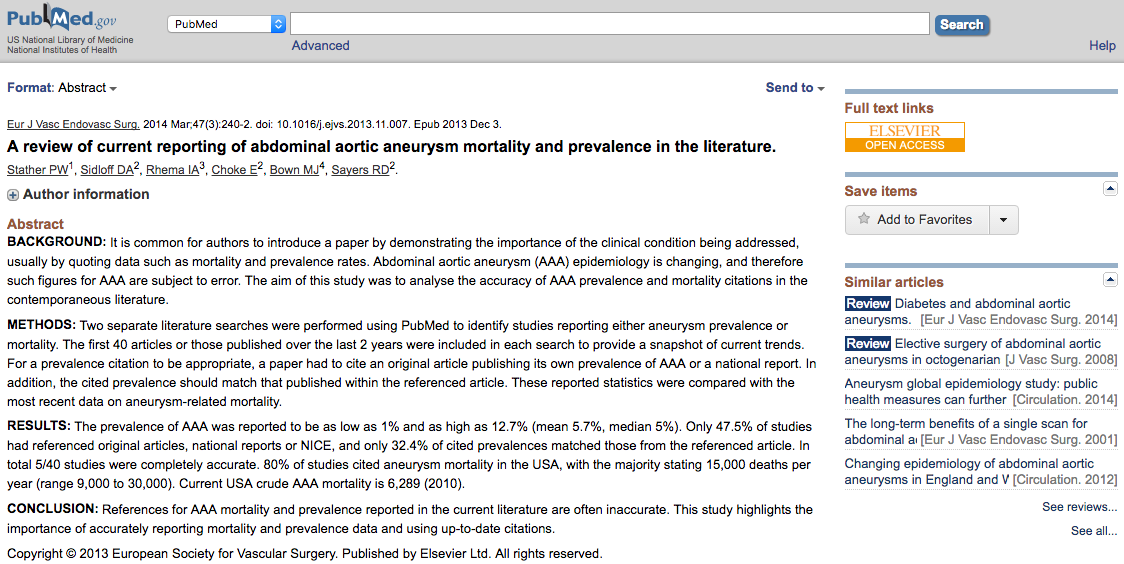Screen capture of the PubMed website displaying an abstract titled "A Review of Current Reporting of Abdominal Aortic Aneurysm, Mortality, and Prevalence in the Literature". The abstract, authored by six co-authors, was published in March 2014 in a journal. The text is structured into the standard sections: Background, Methods, Results, and Conclusion. Additional information includes references and author contact details. The copyright notice states "© 2013 European Society for Vascular Surgery". To the right of the abstract, there are links for full-text access, including one to Elsevier's open-access platform.